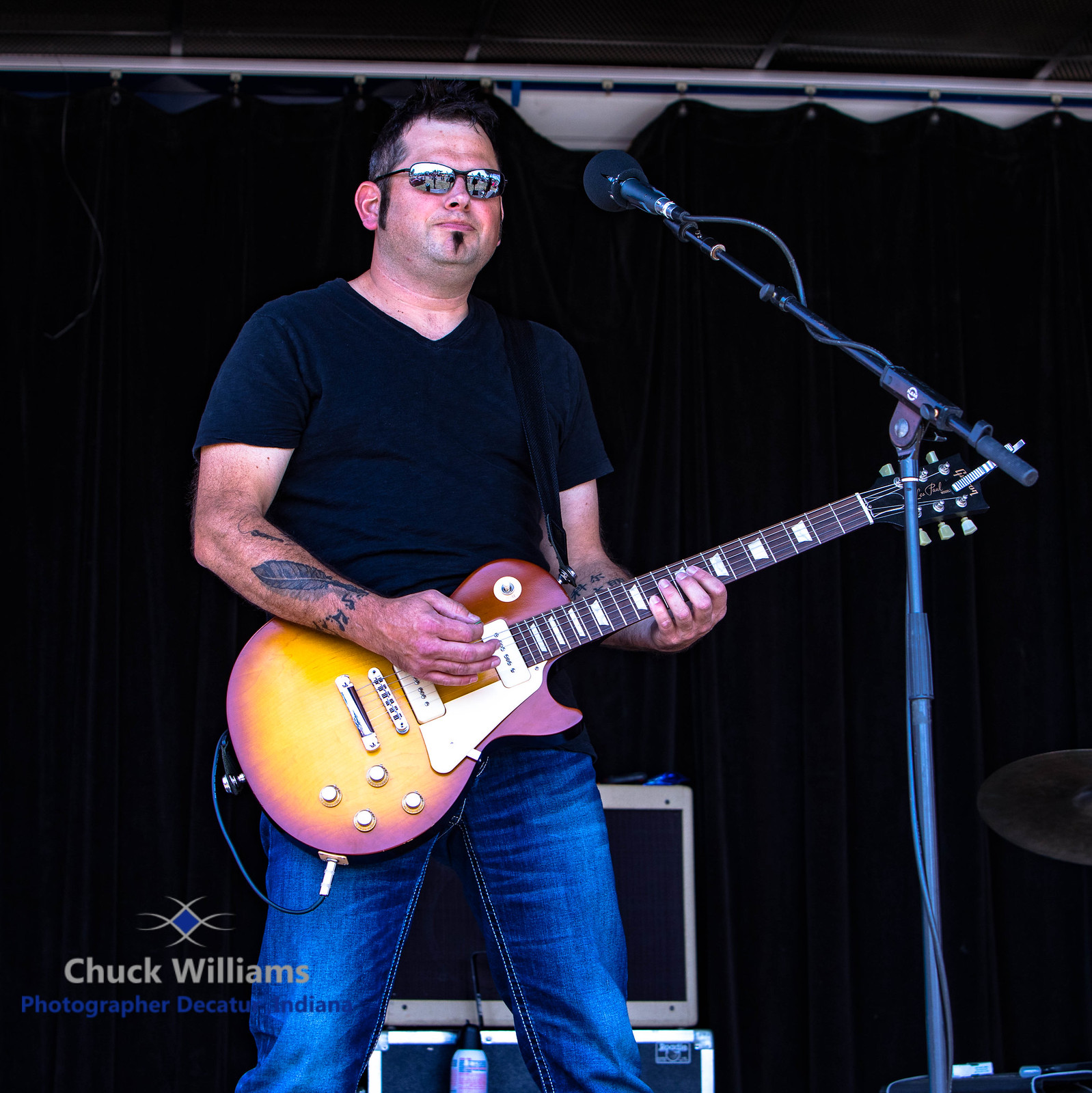The image is a detailed, close-up color photograph of a musician playing an electric guitar at a concert. This white gentleman, who has a short haircut and long sideburns, is wearing dark sunglasses and a V-neck black T-shirt paired with blue jeans. He sports a feather tattoo on his right arm and a distinctive small goatee below his lower lip. The guitar has a striking design with a pinkish to rose-colored outer edge and yellow center. The musician’s left hand is positioned on the guitar's chords while his right hand strums.

Behind him, the stage setup includes two amplifiers and a black backdrop, creating a stark contrast that highlights the performer. A long microphone stretches toward his face, presumably capturing his vocals. In the lower left corner of the photograph is a logo and the partially legible text "Chuck Williams, photographer," followed by something that appears to reference Indiana. The dimensions of the image are roughly six inches wide by seven inches long, indicating a portrait orientation. Overall, the stage setting, musician’s detailed appearance, and equipment are framed meticulously, emphasizing the artistry and atmosphere of the live performance.